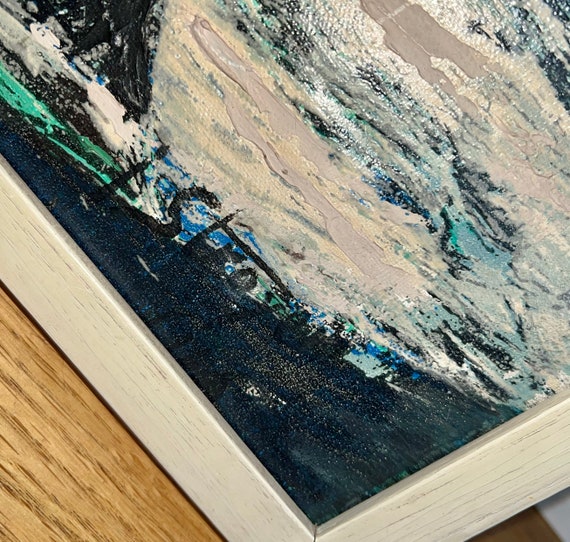The image depicts the bottom right corner of an abstract, surrealist painting framed in a white wood-grain frame, resting on a wooden table. The close-up view focuses on the artist's signature, which appears to be somewhat illegible but includes letters resembling "I-S-T-R-O-Y-E." The painting itself features a complex blend of colors including various shades of blue, turquoise, green, black, white, off-white, cream, and gray, with evident textures where the paint has dried on the canvas. The overall composition of the painting suggests an intricate and expressive use of color and texture, though the specific imagery remains indiscernible.